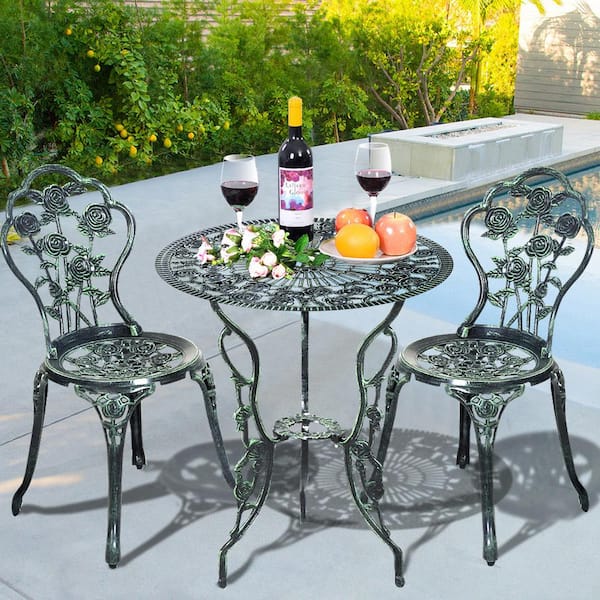A beautifully staged outdoor patio scene featuring a set of two dark green metal chairs and a matching table, positioned on a gray patio floor adjacent to a pool. The chairs, with their Victorian-inspired design, boast intricate rose patterns on the seat and backrest, evident in their stamped metal craftsmanship. The table, standing elegantly on three curvy legs reminiscent of butterfly wings, also showcases ornate rose decorations. Upon the table, two wine glasses filled with red wine and a bottle of wine are carefully placed alongside a plate featuring a selection of fruits—apples and a lemon. The scene is further enhanced by the surrounding lush greenery, dotted with yellow flowers that add a vibrant touch to the background. A large fire pit and the glistening pool contribute to the serene ambiance, while the sunlight, seemingly from a late-afternoon source, casts gentle shadows, suggesting a picturesque setup that might have been artistically modified for a perfect visual harmony.